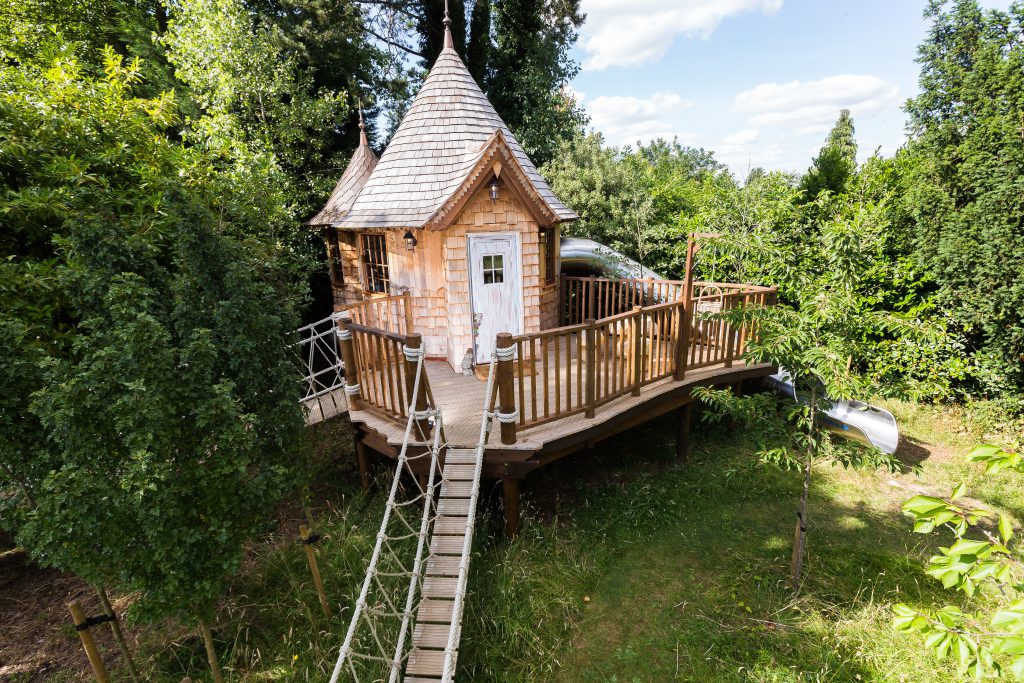In the heart of a lush, forest-like setting, there's an enchanting and whimsical elevated playhouse that exudes a magical charm. Nestled amidst abundant greenery and towering trees, the playhouse stands on sturdy poles, lifting it above the ground. Accessible by heavy-duty rope ladders, the small house features a pointed roof and a welcoming white door, complete with a charming welcome mat. A metal slide extends from the right side of the structure, offering a swift and playful exit. Overhead, the cerulean sky is adorned with scattered, fluffy white clouds, adding to the enchanting atmosphere. This delightful structure, possibly situated in someone's backyard or perhaps a whimsical addition to a forested area, radiates a sense of fun and adventure that appeals to both children and the young-at-heart.